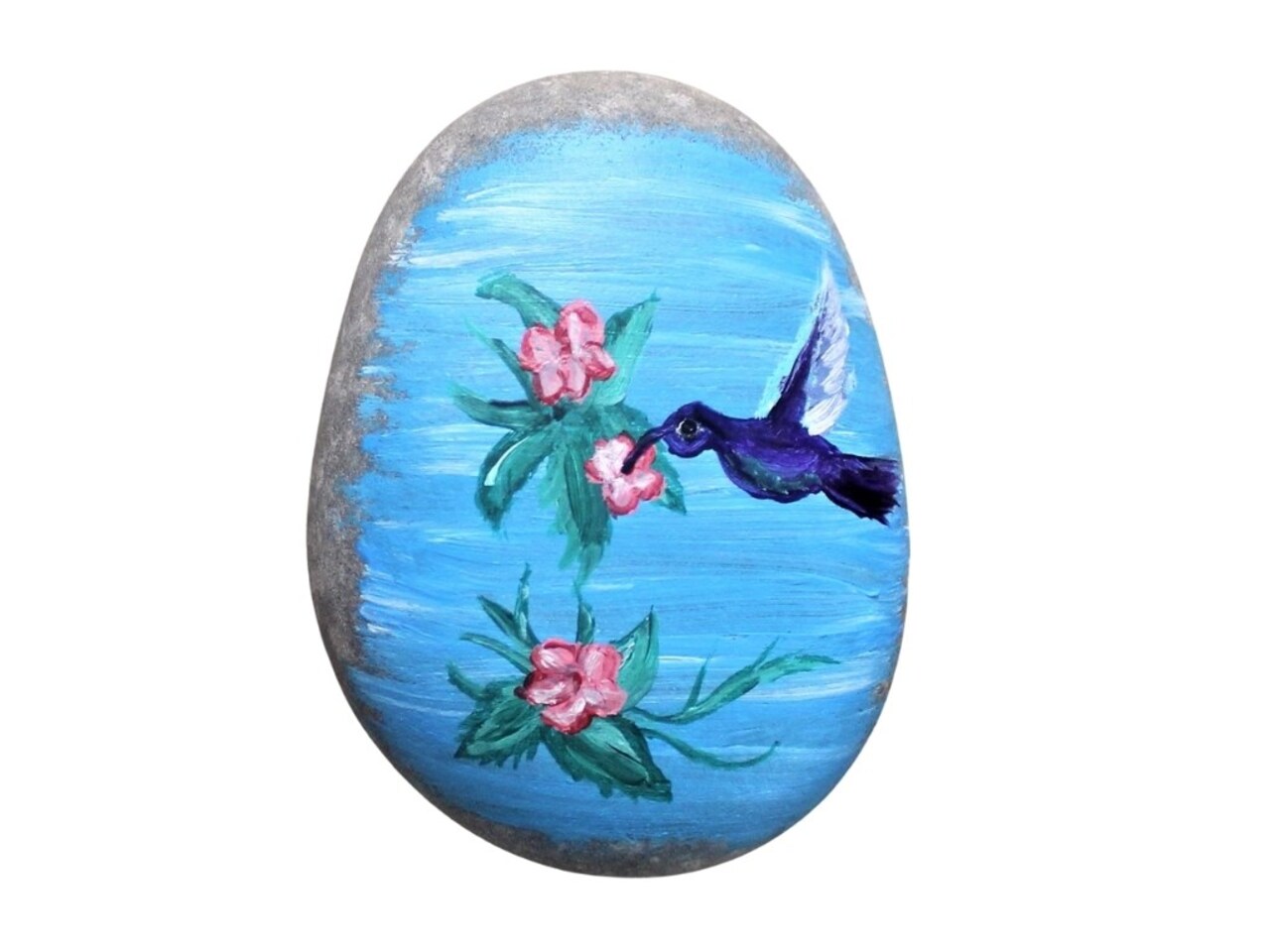The image depicts a smooth, oval-shaped gray rock set against a plain white background. This rock is primarily covered in a painted scene that features sky-blue and white horizontal strokes mimicking the look of a serene sky. Dominating the middle section of the rock on the right side is a detailed, blue hummingbird with white-edged wings. The bird is captured mid-flight, angled towards the left, as it delicately sips nectar from a pink flower. The floral arrangement includes green leaves and three pink blooms, with one flower being attended by the hummingbird and the other two creating a balanced composition below.